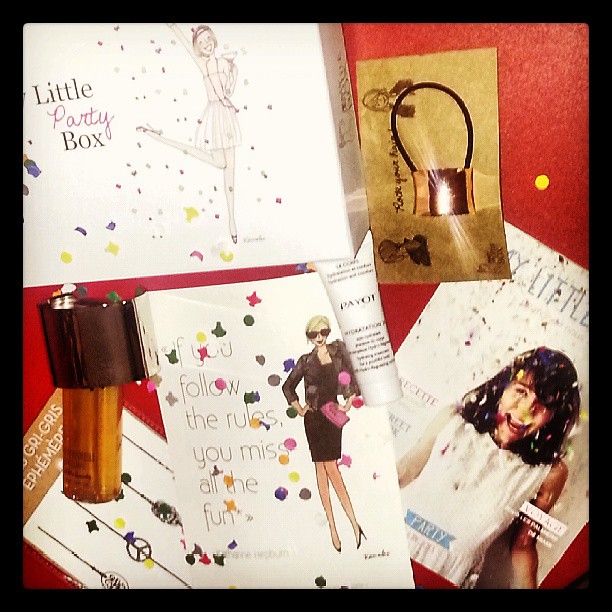This vibrant collage on a red background features a variety of fashion articles, accessories, and festive imagery, centered around the "Little Party Box." In the top left corner, the white box showcases a cartoon woman with one leg up and an arm raised, holding a cocktail, accompanied by the words "LITTLE PARTY BOX" where "PARTY" appears in red and "LITTLE BOX" is in black. To the right, a piece of paper bears the phrase "If you follow the rules, you miss all the fun," with whimsical polka dots surrounding it in green, purple, pink, red, yellow, and orange.

Below the paper, an open magazine depicts a smiling girl among falling confetti, dressed in a black dress and holding a pink bag while wearing black sunglasses. Adjacent to this, a book cover reiterates the same phrase about following rules. Scattered throughout the collage are various products: a white plastic bottle of lotion, a golden bottle with a large brown lid, and what appears to be a can of hairspray resting on a sheet of stickers, one of which displays a peace sign.

To the left, a possible nail polish bottle stands upside down with a gold top. Around it, words like "GREASE" and "EPHEMER" appear in white on a brown background. There's also a slip of paper in cursive, possibly reading "YOUR," flanked by images of people.

Additional items include a black rubber band with a gold locket, bracelets, and more festive polka dots in black, yellow, and blue. The overall composition suggests these elements are part of or inspired by the "Little Party Box," arranged against a rich, celebratory red backdrop.